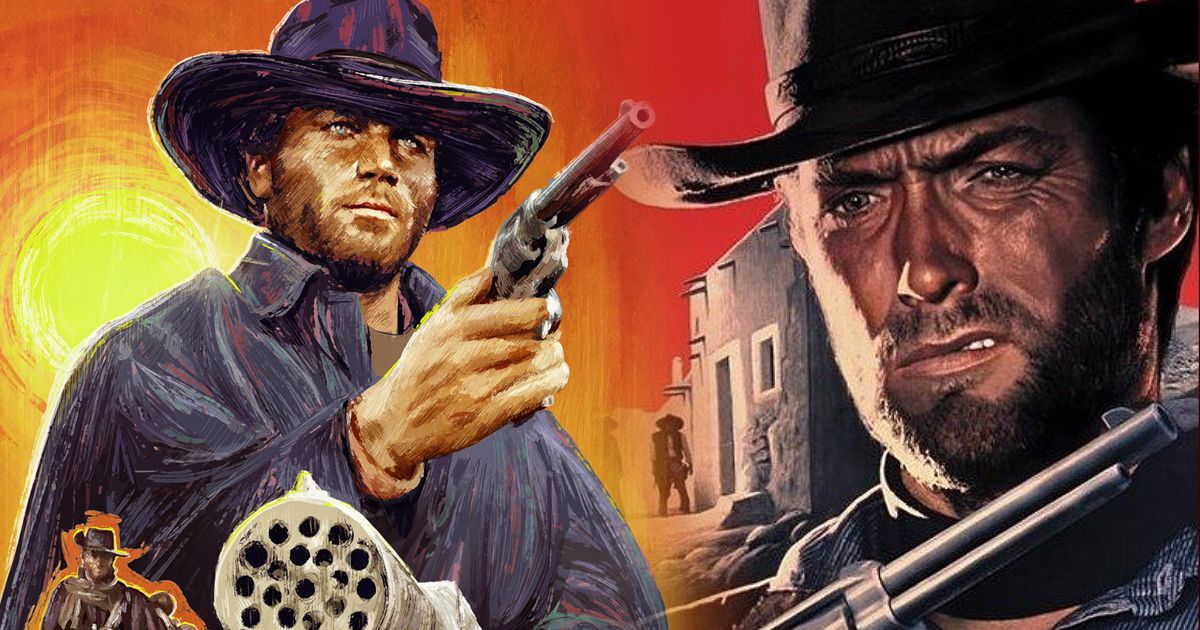This image is a detailed painting or graphic illustration inspired by Clint Eastwood in one of his iconic cowboy roles from a western movie. The landscape-oriented composition features a vibrant color scheme with a striking orange sky and a prominent yellow sun situated in the upper left corner. 

On the left side of the painting, Clint Eastwood is depicted from the chest up, wearing a long dark blue coat and a matching bluish cowboy hat. His right hand is raised, pointing a silver revolver, and he appears to be looking straight ahead with a stern expression. A small orange silhouette rests in the bottom left corner, showing Eastwood again from waist up, clad in a cowboy uniform with a poncho and cowboy hat, reinforcing his tough persona.

To the right of this primary figure, there's an old Wild West style building, grey with a white door frame. In front of the building stands a man in a sombrero, vest, white shirt, and dark pants. In the foreground, the silver barrel of a Gatling gun with many holes is visible, adding an element of intense action.

The right third of the image focuses closely on Eastwood's face. Here, he squints ahead with a determined look, wearing the same cowboy hat. A pistol barrel curves around his neck, emphasizing the western theme. Clint Eastwood is consistently portrayed with a short-trimmed, brownish beard and mustache in all the figures depicted.

Overall, the painting masterfully captures the essence of Clint Eastwood's rugged cowboy image, pairing dramatic visuals with the nostalgia of classic western cinema.